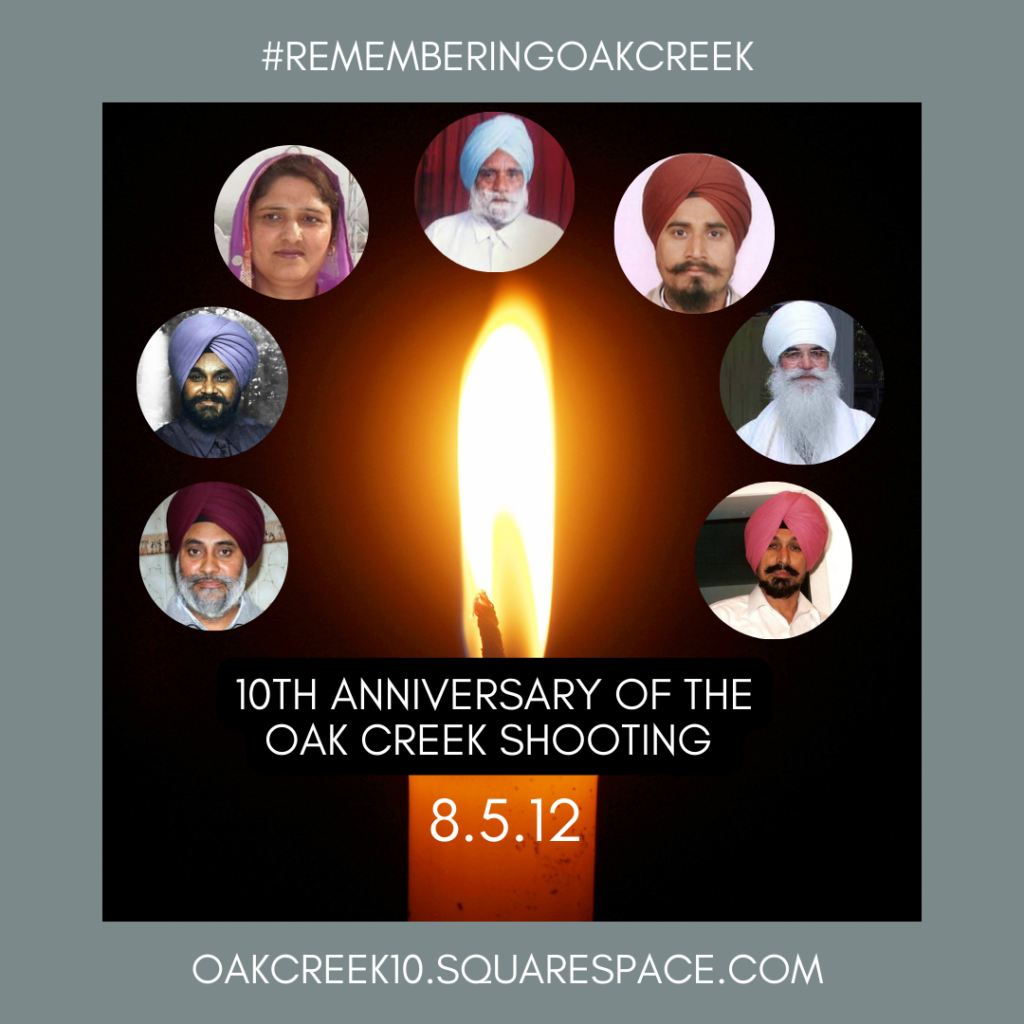A commemorative poster featuring a dark brown and rust brown background with a gray border. At the top of the border, it reads "#RememberingOakCreek" in white lettering. The centerpiece of the poster is a brightly burning candle flame in white, yellow, and orange hues. Surrounding the flame are seven small circles arranged like a clock, each containing the image of an individual, predominantly men wearing Sikh turbans and one woman with a colored veil, all of dark complexion, indicating they are of the Sikh faith. Below the flame, within the brown section, it reads "10th Anniversary of the Oak Creek Shooting" in white text, and on the orange rust-colored candle base, it states "8.5.12." At the bottom, the text "oakcreek10.squarespace.com" is prominently displayed.